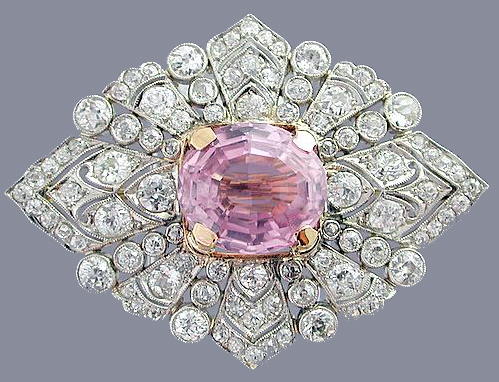The image is a professionally staged, full-color, square photograph of an intricate piece of jewelry set against a light blue background. The central focus of the piece is a large, intricately cut purple gemstone, possibly an amethyst, encased in a gold frame. This gemstone is square-shaped with its top four corners secured by gold elements. Surrounding the central stone are numerous small, white jewels arranged in circular patterns that extend outward, creating a diamond-like shape with a sunburst design. The outer edges of this pattern have larger points at the top, bottom, left, and right, enhancing the overall diamond visualization. The entire piece is lavishly detailed, showcasing white or silver elements, possibly white gold or silver, that add to the luxurious presentation of the jewelry.